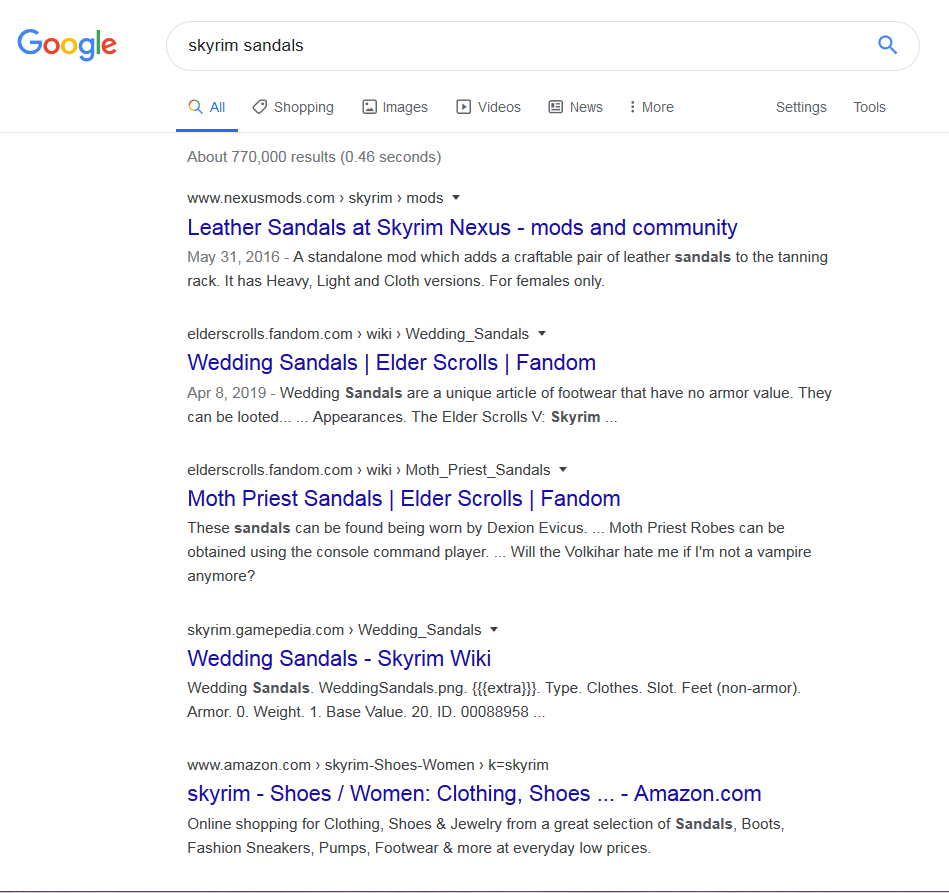The image depicts a Google search results page. In the upper left corner, the Google logo is prominently displayed. To the right of the logo is the familiar white search bar, accompanied by a blue search icon on its right end. Inside the search bar, the query "Skyrim Sandals" is clearly typed out. Beneath the search bar, there's a row of selectable tabs labeled "All," "Shopping," "Images," "Videos," "News," "More," "Settings," and "Tools." Just below these tabs, the search results information is shown, indicating approximately 770,000 results retrieved in 0.46 seconds.

The first search result is from nexusmods.com, titled "Leather Sandals at Skyrim Nexus." Next is a link to "Wedding Sandals" on the Elder Scrolls Fandom site, followed by "Moth Priest Sandals," also on the Elder Scrolls Fandom site. The fourth search result is "Wedding Sandals" on the Skyrim Wiki. The final highlighted website is an Amazon listing, described as "Skyrim-shoes-womenclothingshoes-amazon.com."